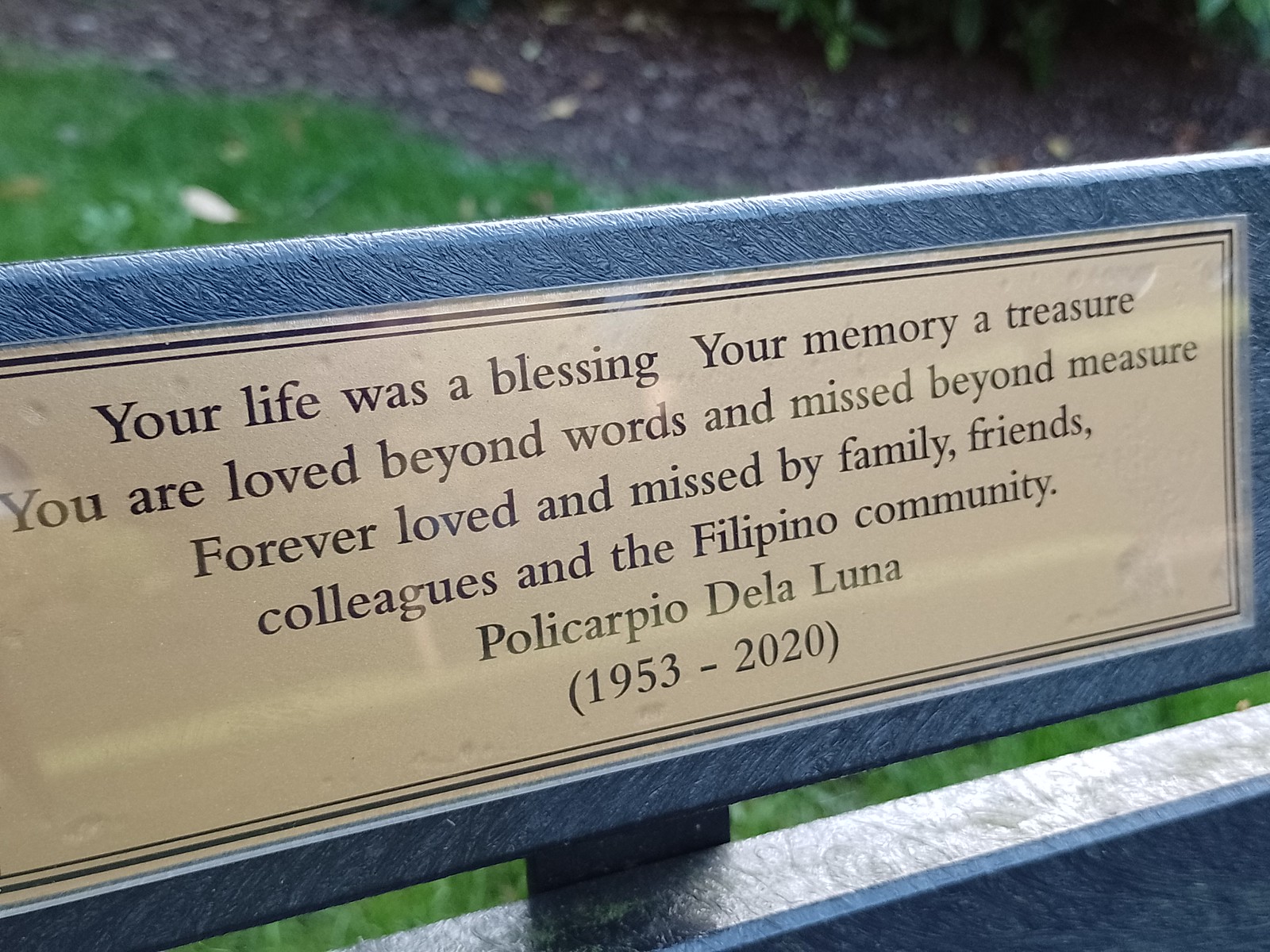In the image, there is a golden plaque mounted on what appears to be the back of a bench, elevated with another bench part below it. The plaque carries an inscription in dark brown text over a light tan background, which reads: "Your life was a blessing, your memory a treasure. You are loved beyond words and missed beyond measure. Forever loved and missed by family, friends, colleagues in the Filipino community." Below the inscription, it names Polycarpio de la Luna (1953-2020). The bench is situated in a well-kept area, possibly a cemetery or park, as indicated by the neatly mown grass and darker brown soil with scattered leaves and nearby shrubs and trees. The plaque has a gray border with black lines of increasing thickness around it.